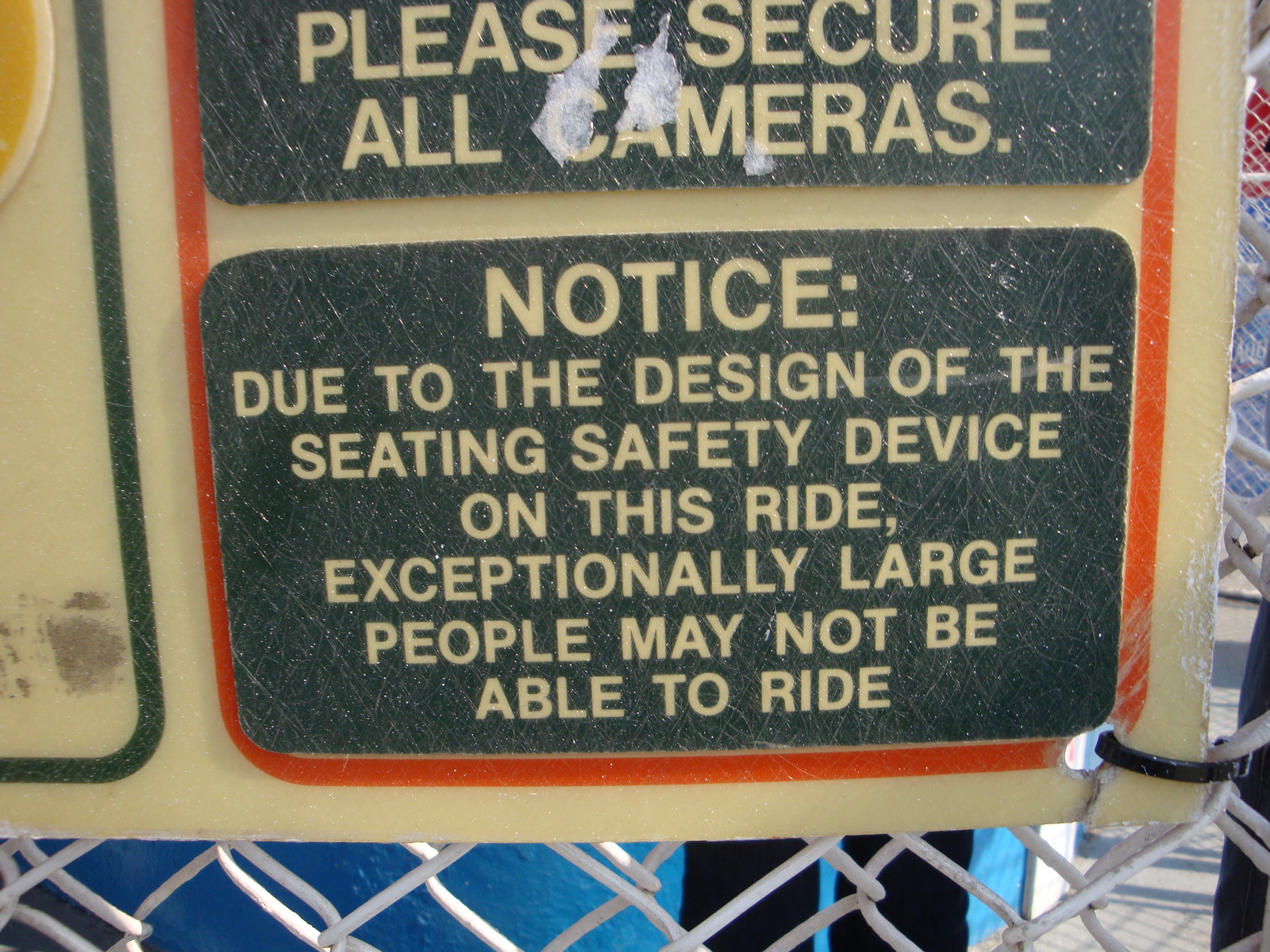This photograph, taken during the daytime, captures a weathered sign affixed to a white chain link fence at an amusement park, presumably at the entrance to a ride. The sign, featuring a yellow background with black rectangular areas and a rounded orange border, is secured with black zip ties and has a somewhat beat-up appearance, indicating it has been there for a while. The upper part of the sign partially visible, reads, "Please secure all cameras." Below it is a more detailed notice in white text: "Notice: Due to the design of the seating safety device on this ride, exceptionally large people may not be able to ride." This warning is clearly intended for those standing in line for the ride. Additionally, the left side of the sign shows a black border, suggesting there is more information that is out of the frame. Enhancing the sign's text clarity are green and orange outlines. Overall, the detailed message reinforces safety measures for the amusement park’s visitors.